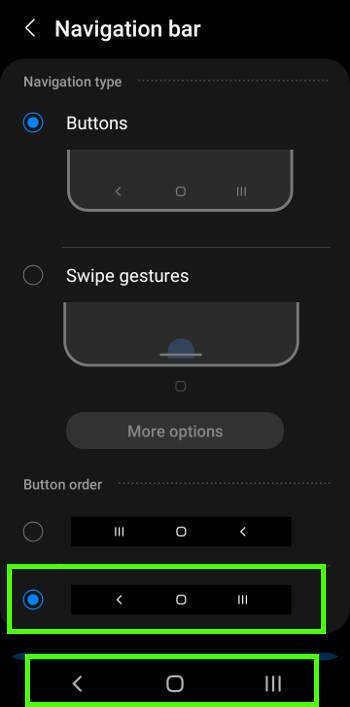The image features a user interface screen with a predominantly black background at the top. At the very top of the image, there's a navigation bar containing a white left arrow. Below this bar, a black box labeled "Navigation Type" indicates "Buttons," accompanied by a blue circular button next to it. 

Progressing downwards, there's a light gray box containing various icons: a left arrow, a circle, and three horizontal lines. Adjacent to this, another option labeled "Swipe Gestures" is marked, with a corresponding circular icon.

Following this, another light gray box presents a light blue circle with a line extending from it, leading to a small central circle icon. Just below, a gray box labeled "Button Order" displays a small circle and another black square containing three lines, a square, and a left arrow.

At the bottom, two options, outlined in green, are visible. The first, highlighted with a blue button, includes the icons for a left arrow, the box, and three lines. Similarly, the second green-outlined option also displays a left arrow, a box, and three lines.